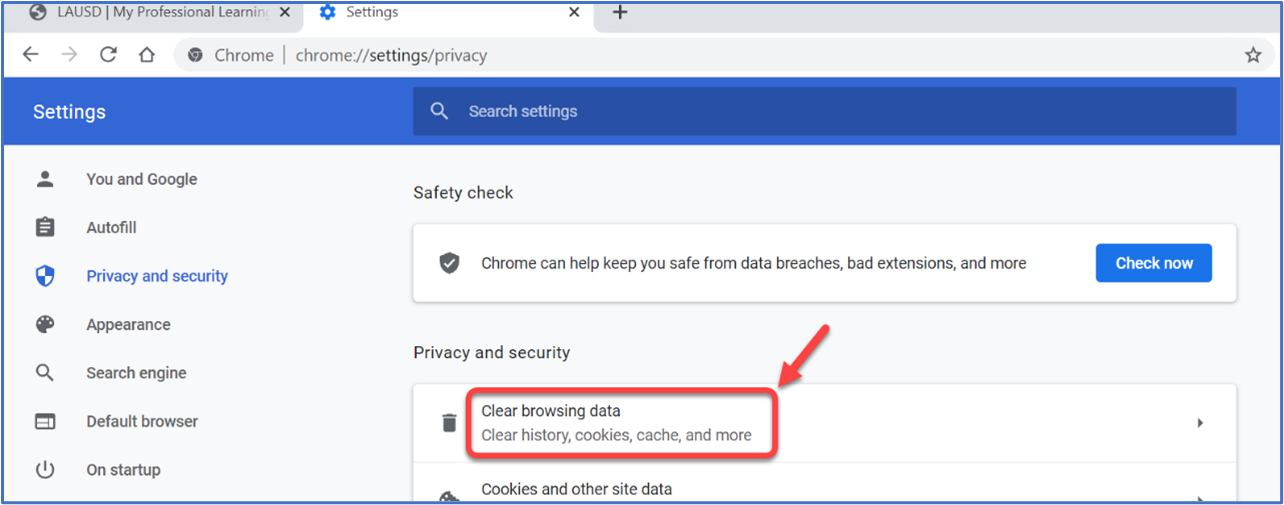The image shows a computer screen open to the settings page of the Google Chrome browser. At the top left corner of the screen, there's a label that says "LAUSO / My Professional Learning" followed by another tab labeled "Settings".

On the main settings page, the URL bar displays "chrome://settings/privacy". The left side of the screen features a vertical menu with various settings categories, including a search bar labeled "Search settings". The main categories listed horizontally in this menu are: "You and Google", "Autofill", "Privacy and Security", "Appearance", "Search Engine", "Default Browser", and "On Startup".

On the right side of the screen, there is a section titled "Safety Check" with a brief description: "Chrome can help keep you safe from data breaches, bad extensions, and more". There is also a "Check now" button.

Below the "Safety Check" section, the "Privacy and Security" category is displayed. A red rectangle outlines a specific option named "Clear browsing data", which includes descriptions like "Clear history, cookies, cache, and more". An adjacent icon of a garbage can symbolizes the clearing action. A detailed red arrow points to this outlined section to draw attention.

Underneath "Clear browsing data", there is another option labeled "Cookies and other site data". This option is displayed in a white box with black text, with arrows on the right side indicating that it can be clicked for more options.